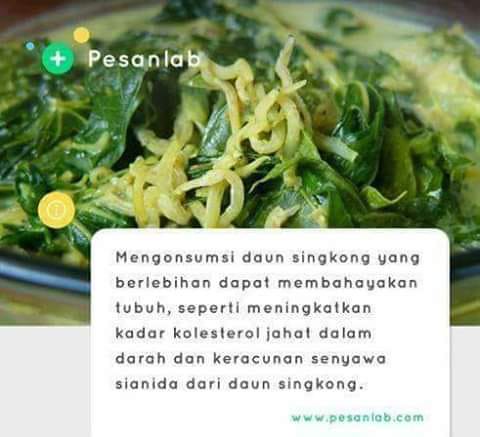This photograph showcases a vibrant, green salad dish featuring spinach-like leaves interspersed with yellow vegetable strands, artfully arranged on a blue plate. The top left of the image contains a green circle with a white plus symbol alongside white text that reads "Pisan Lab." Below, a small yellow circle with a white informational 'I' symbol is visible. A notable white rectangle with rounded edges at the bottom of the image contains text in another language, starting with "MENGONSUMSI DAUN SINGKONG." The lettering suggests this may be a Southeast Asian or possibly a Korean dish. The overall scene is suggestive of an informational snapshot, likely from a website or recipe page, providing details about the dish and its nutritional benefits.